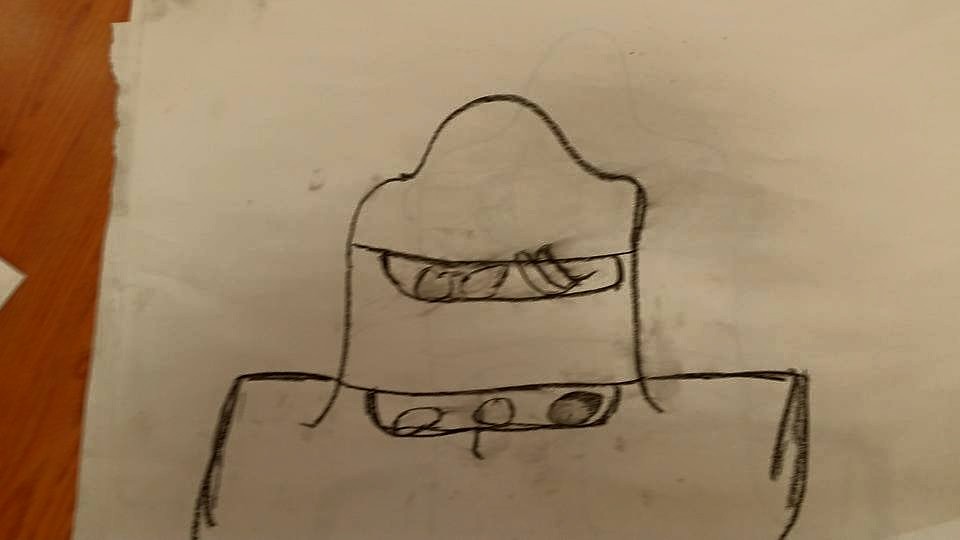The image is a digital photo capturing a child's drawing on a piece of white paper, which is slightly off-center to the left. The paper rests on a nicely grained brown wood floor, featuring darker and lighter shades of tan. The drawing itself appears to be done with a black crayon or pencil, given some smudging and areas that seem heavily shaded or altered.

The central figure in the drawing resembles a robot with notable details. The "head" of the robot has a distinct shape with three lumps: one at the top and two on the sides, creating a non-round appearance. Below the head, a line suggests a brow, and beneath that, a slit likely represents the eyes, similar to a visor. The structure directly under this is a rectangular section, resembling a breastplate. Both at the top middle of this rectangle and at the bottom, three circles are drawn, with the right-side bottom circles being more heavily colored in.

Overall, the marks on the paper indicate significant erasing and redrawing, highlighting the child's effort and adjustments while creating this robotic figure.